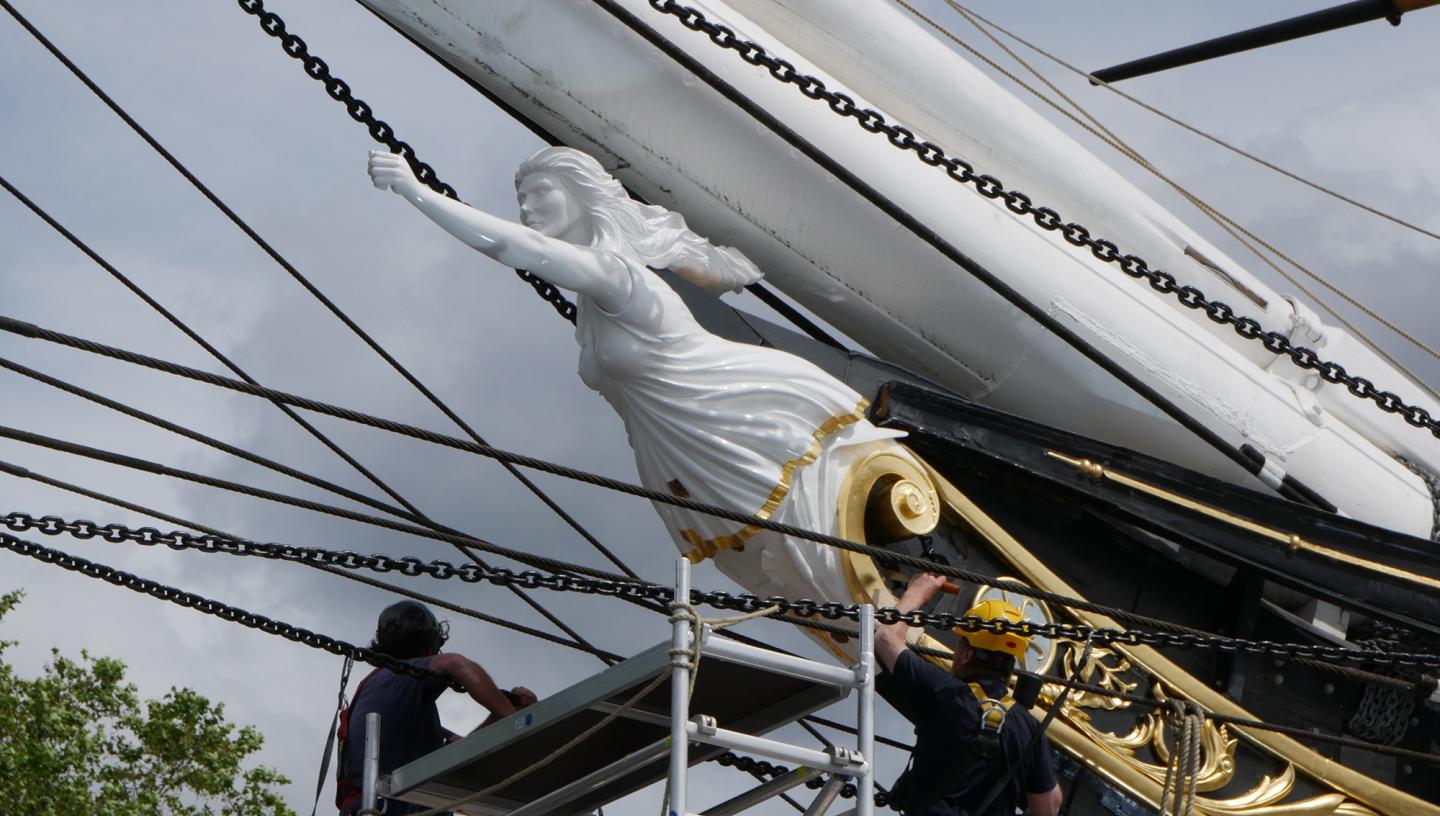In this photograph, taken outside on a stormy, gray day, the close-up view reveals the bow of what is likely the USS Constitution, characterized by its black hull with intricate gold trim and white accents. Prominently featured at the front is the impressive white statue of a lady, possibly made of stone or marble, with long flowing hair cascading behind her and an elegant dress adorned with gold etchings at the hem. The statue's left arm is outstretched in a fist raised forward, pointing towards the horizon. Surrounding the statue are numerous ropes and black chains, as well as a large white circular tube that could be part of the ship's rigging.

Below the statue, two construction workers are engaged in restoration work. One worker, standing on scaffolding and wearing a yellow helmet, is seen painting part of the black hull. Another sits or stands on additional scaffolding on the opposite side. The ship appears meticulously maintained, with the black, white, and gold elements in pristine condition, suggesting ongoing preservation efforts. In the background, a hint of green from a tree is visible, further indicating that the ship is on land undergoing restoration.